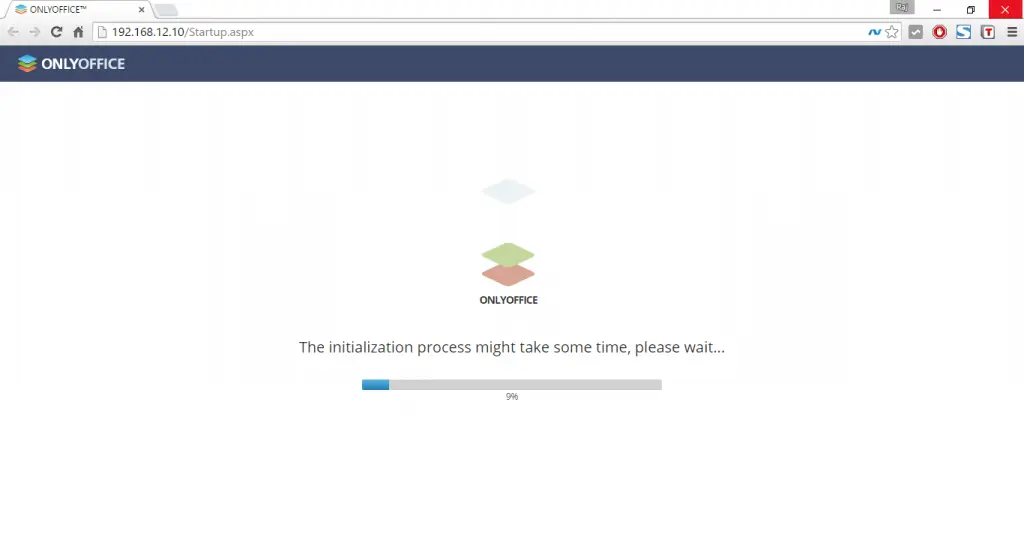In the image, a computer screen displays a web browser tab labeled "OnlyOffice." The browser's search bar contains the URL "192.168.12.10/Startup.aspx," entered in lowercase. To the right of the search bar, a star icon signifies a bookmarking feature. Adjacent to this, several browser extension icons are visible: an unknown grayed-out extension, a stop sign symbolizing an ad blocker, a white "S" on a blue background, and a red "T" on a white background. Further to the right, the browser's settings icon, represented by three horizontal bars, is visible.

The main section of the webpage features the OnlyOffice logo with an installation progress message below it. The message reads, "The installation process might take some time. Please wait," and the current installation progress is at 9%.